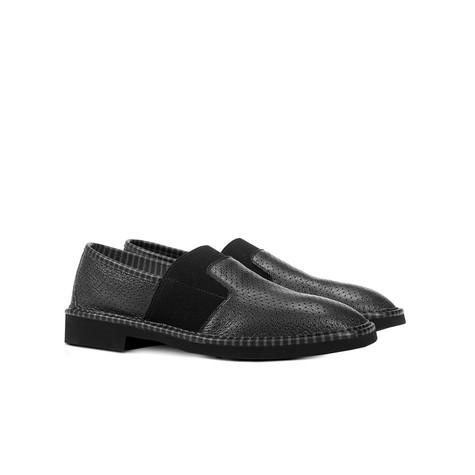In this image, there is a pair of black leather loafers positioned at a diagonal angle against a completely white background. The shoes, facing towards the right, are slip-ons with no laces, featuring a stretchy elastic section where the laces would typically be. They have small, intricate holes for breathability and are detailed with prominent stitching all over the leather surface. Each shoe has a small heel and a flat bottom, emphasizing a somewhat formal, dressy appearance. The detailed texture of the leather, along with the solid black, off-black, and gray hues, makes the shoes stand out against the blank background, suggesting it is a product image akin to those seen in online shoe stores.